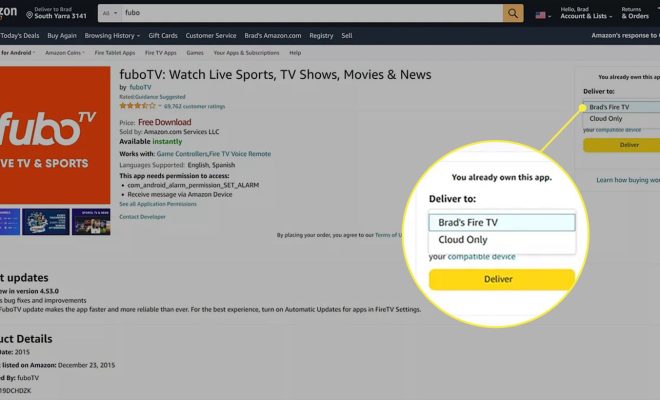**Image Description: Amazon Product Page for FuboTV**

The image displays a portion of an Amazon product page specifically for FuboTV, a streaming service offering live sports, TV shows, movies, and news. The main feature of the product listing is a prominent orange-red box with the text "FuboTV" in white. To the right of this box, the text "Buy FuboTV" is visible, indicating the app is available for free download, which is highlighted in red text.

Details reveal that the app is sold by Amazon.com Services LLC and is available for instant download. The app is compatible with game controllers, player TVs, and voice remotes. It supports multiple languages including English and Spanish. There is also a note that the app requires permissions to access certain functionalities on the Amazon device, including the ability to receive messages.

Additional information about updates and service details is visible in the text on the page. On the right side, there is a specific section that appears to magnify certain content, showing a close-up view. This magnified view indicates a message stating "You already own this app" and offers options to deliver the app to either "Brad's Fire TV" or "Cloud Only". Below this, there is a note about the compatibility of the device and a yellow button labeled "Deliver".

Overall, the image captures comprehensive information about the FuboTV app, highlighting its availability, features, and delivery options on the Amazon platform.